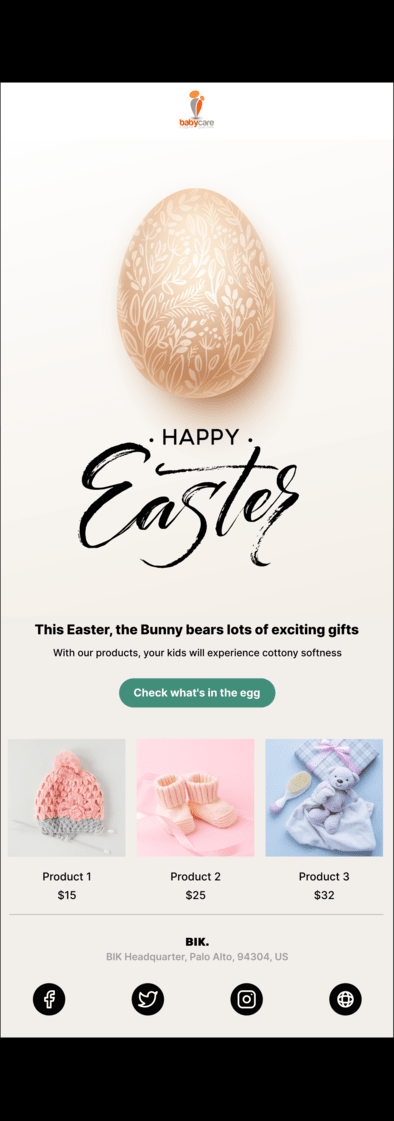**Detailed Caption:**

The image is a screenshot of a mobile app or website promoting baby care products. At the top, the app's header reads "Baby Care Baby's Orange Care" in gray text. Below this, there is an intricately designed, pinkish Fabergé-like egg with a floral pattern that resembles wallpaper. Just beneath the egg, in bold black letters, the text "Happy Easter" is displayed. 

Further down, a black font message reads: "This Easter, the bunny bears lots of exciting gifts. If you like our products, comment your kids will experience cotton softness." Beneath this message is a green button with white text that says, "Check what's in the egg."

Following the button, there are three images arranged horizontally. The first image on the left showcases a pink baby beanie with a gray border, labeled as "Product 115" and priced at $15. The second image in the middle displays a pair of pink baby booties adorned with a pink bow, labeled as "Product 200" with a price of $25. The third image on the right features a collection of baby items: a small teddy bear, a baby brush, a spit-up bib, and a flannel cloth with a pink bow, labeled as "Product 300" and priced at $32. All of these items predominantly feature purple and pink hues.

At the bottom of the screenshot, the text "BIK" is written in black letters, followed by the location details: "BIK headquarters, Palo Alto, 94304 US, including California."